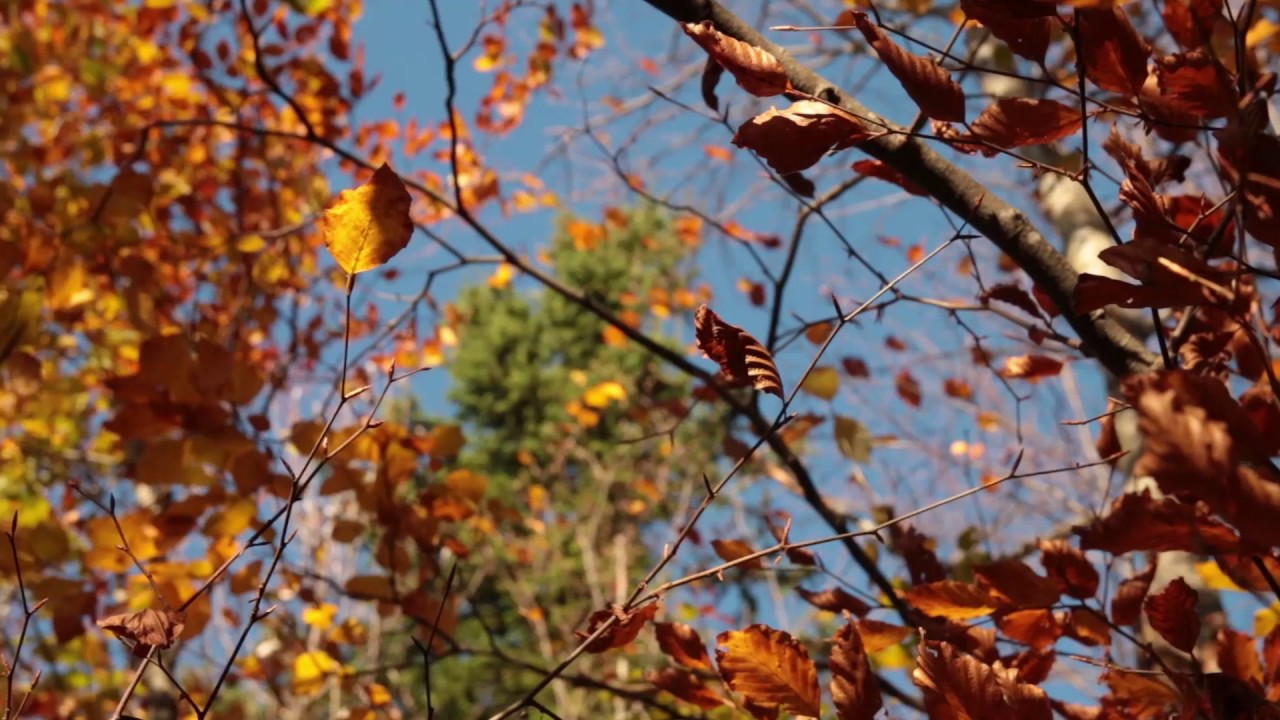The photograph, taken on a sunny day, offers a detailed, close-up view looking upwards through the sparse branches of a foreground tree, where autumn's vivid colors are on display. The branches, medium in diameter and grayish-brown, occupy the right side of the image. Several leaves cling to these branches, displaying a spectrum of fall hues—reddish, orangish, and brownish. A point of focus in the image is a thin twig with a small, brownish bug of indeterminate species, about a couple of inches long, adding a touch of life to the stillness.

In the background, the sky is a clear, vibrant blue, devoid of clouds and illuminated by bright sunlight, enhancing the colors of the foliage. To the left, another tree emerges with dense, golden-brick colored leaves, accented by a few bright yellow leaves towards the center. The background also features a much larger tree with predominantly green leaves, presenting a stark contrast to the autumnal colors of the surrounding trees. This richly detailed scene captures the essence of early fall in a countryside setting, where the changing seasons paint a vivid tapestry of colors against the backdrop of an unmarred blue sky.